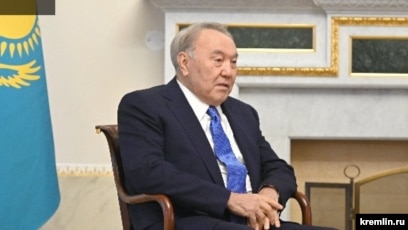The image depicts an older man with short gray hair and a receding hairline, sitting in a brown wooden armchair. He is attired in a dark blue or navy suit with a blue tie and a white button-down shirt. His hands are resting atop one another in his lap, and he is gazing off to the right. The background features a gray wall alongside a white or beige wall with gold trim and a decorative pattern, as well as a mantle and a fireplace area. Behind the man, there is a blue and yellow flag displaying a sun and wing motif. The floor appears to be covered in light tan tiles. In the bottom right corner, a small black box with white text reads "Kremlin.ru." This horizontally aligned, low-resolution rectangular image seems to be a frame from a video.